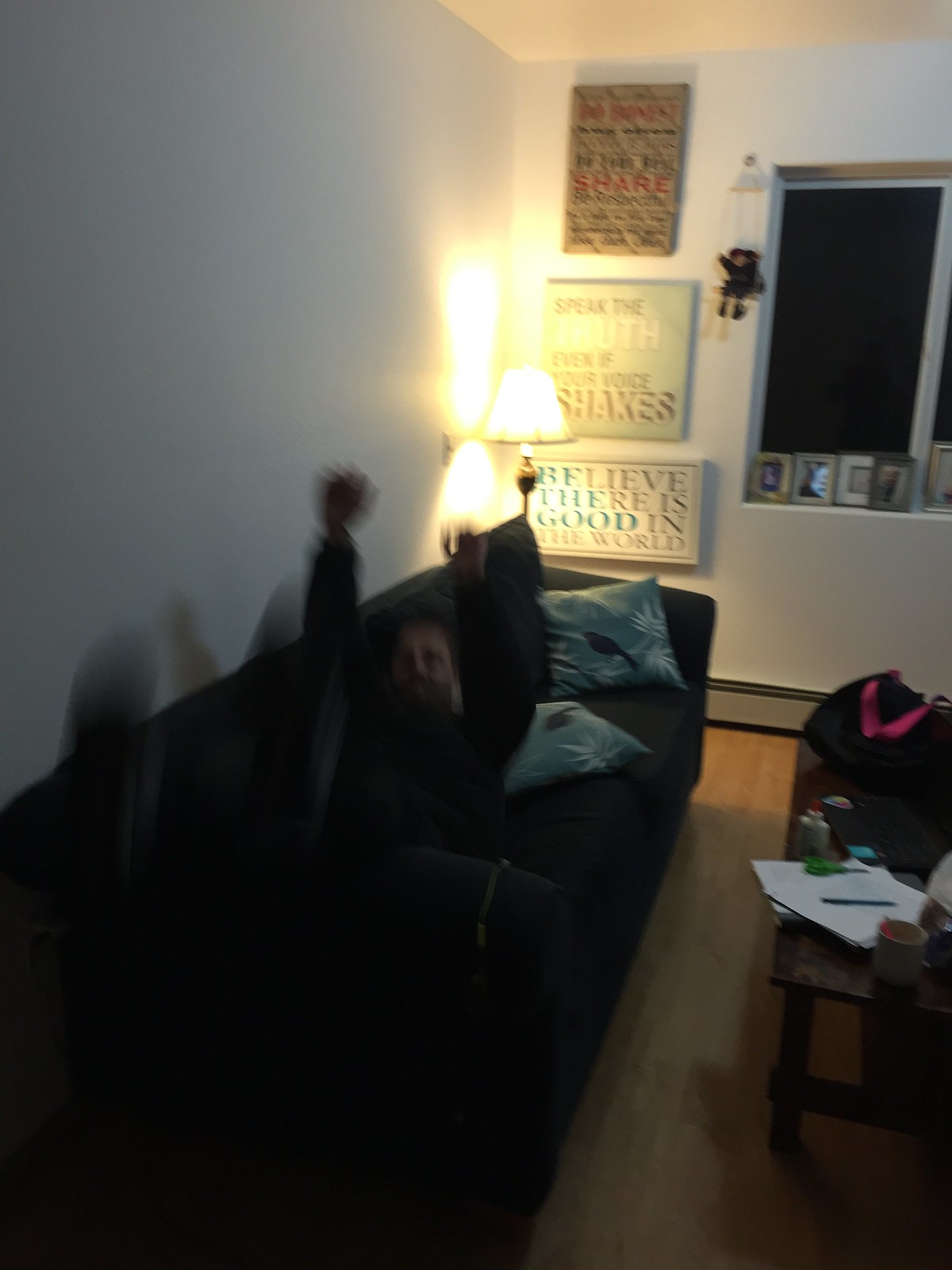This slightly blurry image captures a dynamic scene within a cozy, dimly lit living room. In the foreground, a man, dressed in an all-black outfit, appears to be mid-fall onto a black couch that is adorned with two blue pillows, detailed with black birds and white flowers. His arms are raised, possibly in the act of catching himself, but the motion gives his figure a blurred appearance. Adjacent to the couch is a small coffee table cluttered with an assortment of items, including a mug, papers, a pen, an Elmer's glue container, arts and crafts supplies, a laptop, and a black duffel bag with pink straps.

The room's walls are decorated with an array of art and motivational quotes. Prominently, placards display phrases like "Believe there is good in the world" and "Speak the truth, even if your voice shakes." Below these inspirational messages are additional picture frames. To the left hangs a small toy or puppet suspended by strings. 

The far side of the room features a window, enveloped in darkness, providing no outside view. Framed photos rest on the windowsill. The ambient light source, likely a lamp in the corner of the room, casts deep shadows that emphasize the cozy yet cluttered atmosphere of the space.